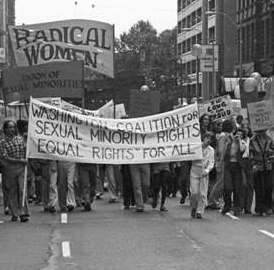This is a small, square, black-and-white photograph capturing a historic protest march in a city. The image, though old and grainy, vividly depicts a crowd of predominantly men walking down the street, holding various signs and banners. The focal point is a large banner at the front, held aloft by two people, with the text "Washington Coalition for Sexual Minority Rights: Equal Rights for All." Further back, another prominent sign reads "Radical Women." The procession is flanked by city buildings and tall trees, enhancing the urban backdrop. Although many protesters bear smaller signs, the text on them is difficult to decipher due to the photo's resolution.